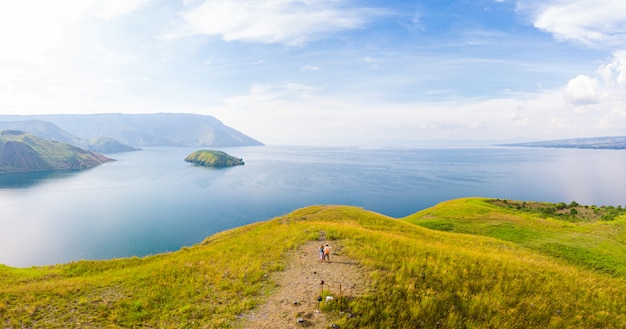The photograph captures a breathtaking outdoor scene featuring rolling grassy hills in various shades of green, interspersed with hints of tan and yellow. These hills slope gently towards the edge of a vast, bright blue body of water, presumably a lake or sea. A dirt or gravel pathway, clear of grass, leads up to the edge where two tiny figures—a couple with one person in a pink top and another in a blue or orange top—stand, gazing out at the magnificent, serene view. The expansive water, which stretches out to the horizon and reflects the scattered wispy white clouds in the blue sky, is bordered by additional landmasses: a larger one to the left and a small green island towards the center. Far off in the distance, hazy mountains are faintly visible, adding depth to the landscape. The vibrant, sunny ambiance and the beauty of nature make it an inviting and peaceful scene.